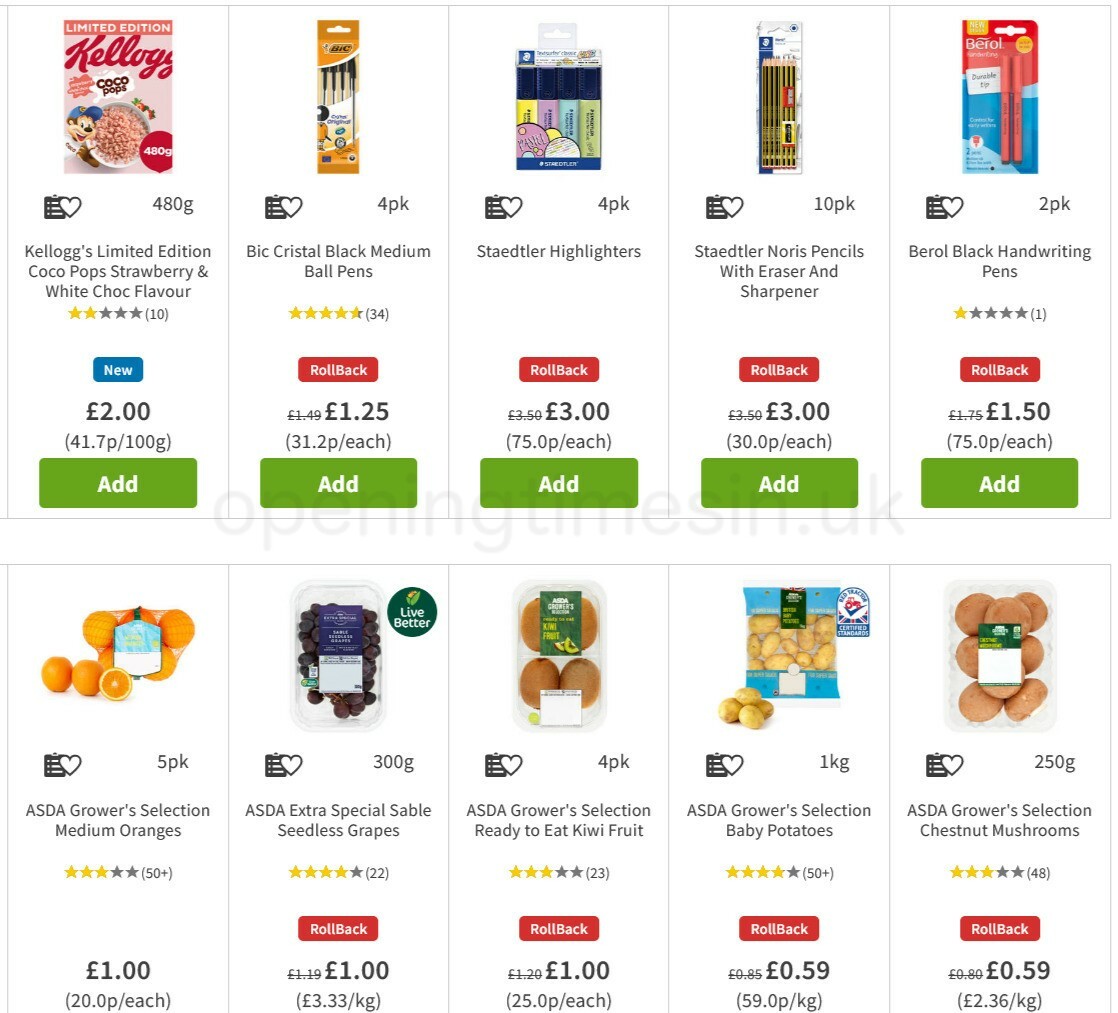The screenshot depicts a section of an e-commerce website with a clean, white background. The page is structured in approximately two rows, with each row containing five product images framed by thin, gray borders. Each product listing includes a detailed image and a consistent format for presenting product information.

**Top Row:**
1. **Kellogg's Limited Edition Cocoa Pops Strawberry and White Choco Flavor**:
   - Image of the Cocoa Pops product.
   - User rating: 2 out of 5 stars, based on 10 reviews.
   - Blue "New" label.
   - Price: £2.00.
   - Cost per unit weight: 41.7p/100g.
   - Green "Add" button for adding the item to the cart.

2. **Big Crystal Black Medium Ball Pens**:
   - Image showcasing a package of ball pens.
   - Similar detailed layout for pricing and user interaction.

3. **Staedtler Highlighters**:
   - Image of highlighters in their packaging.
   - All pertinent item details in accordance with the consistent formatting.

4. **Staedtler Norris Pencils with Eraser and Sharpener**:
   - Product image featuring a package of pencils, an eraser, and a sharpener.
   - Consistent user interface elements as outlined in the format.

5. **Daryl Black Handwriting Pens**:
   - Image of the handwriting pens package.
   - Includes all standard details such as price, reviews, and interaction buttons.

**Bottom Row:**
1. **ASDA Grower's Selection Medium Oranges**:
   - Image of a pack of medium-sized oranges.
   - Includes details on pricing, reviews, and add-to-cart options.

2. **ASDA Extra Special Sable Seedless Grapes**:
   - Product image of seedless grapes.
   - All necessary product information presented similarly to other items.

3. **Ready to Eat Kiwi Fruit (ASDA)**:
   - Image featuring ready-to-eat kiwi fruits.
   - Consistent with the format of detailed product description and purchasing options.

4. **Baby Potatoes (ASDA)**:
   - Photo of a package of baby potatoes.
   - Follow standard information presentation for ease of user navigation.

5. **Chestnut Mushrooms (ASDA)**:
   - Product image of chestnut mushrooms.
   - Situated in the bottom right corner, complete with all standard details.

Each product listing on this e-commerce site seamlessly integrates an image, user reviews, a price breakdown, cost per unit weight, packaging weight, and convenient buttons for adding items to the shopping cart. This organized format enhances the user experience by providing clear and concise information for informed purchasing decisions.